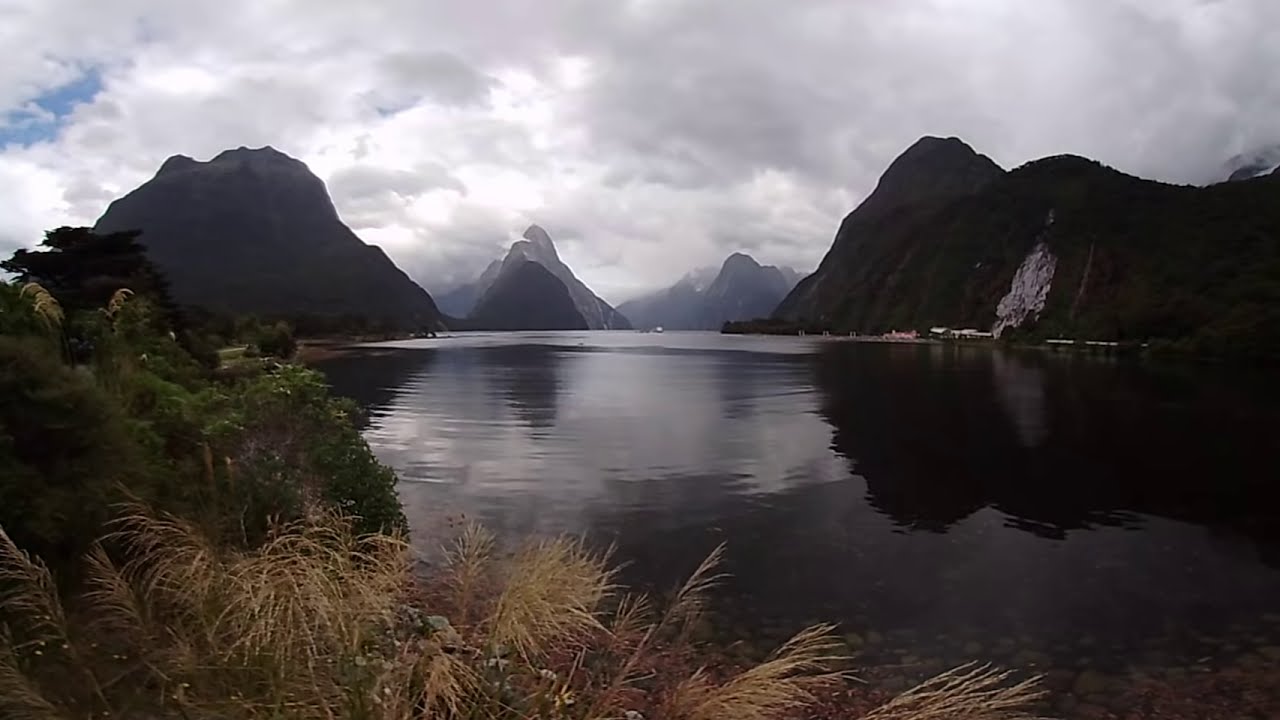This image captures a serene and picturesque nature scene featuring a calm lake surrounded by scenic, snow-dusted mountains or large hills. The sky overhead is predominantly covered by thick clouds, with only small patches of blue sky visible. The lake water is remarkably still, with gentle ripples and a clear reflection of the mountains. In the foreground, there are some tan-colored, skinny plants and green leaves from trees on the left, along with some visible gravel beneath the shallow parts of the water. While no fish or wildlife can be seen, there are hints of human activity in the distance, with small boats and piers suggesting possible recreational use. The overall setting is peaceful and beautifully captures the essence of untouched nature.